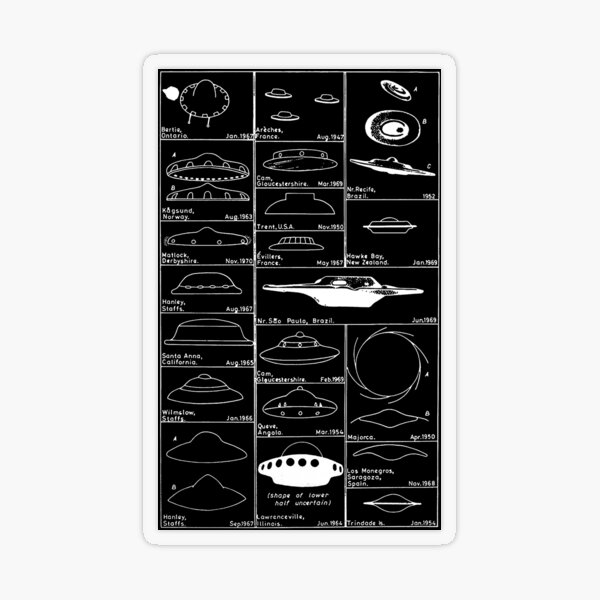This image features a detailed chart showcasing various types of flying saucers or UFOs, set against a black background with white sketches. The chart includes approximately three to four distinct saucer shapes, each identifiable by their unique styles yet sharing common design elements such as a thicker bottom or middle section and a thinner top part. Notably, the flying saucers are divided into multiple parts, illustrating different descriptions. The top left saucer resembles a Mexican sombrero, while the top right features a Frisbee-like shape with an indentation. Other depicted saucers range from dome-shaped to flat, including those with domed tops. Each UFO is meticulously sketched, along with annotations listing the cities where they were reported, spanning various global locations such as Birdie, Ontario; Kingsund, Norway; Matlock, Derbyshire; Santa Ana, California; and near Sao Paulo, Brazil, among others.